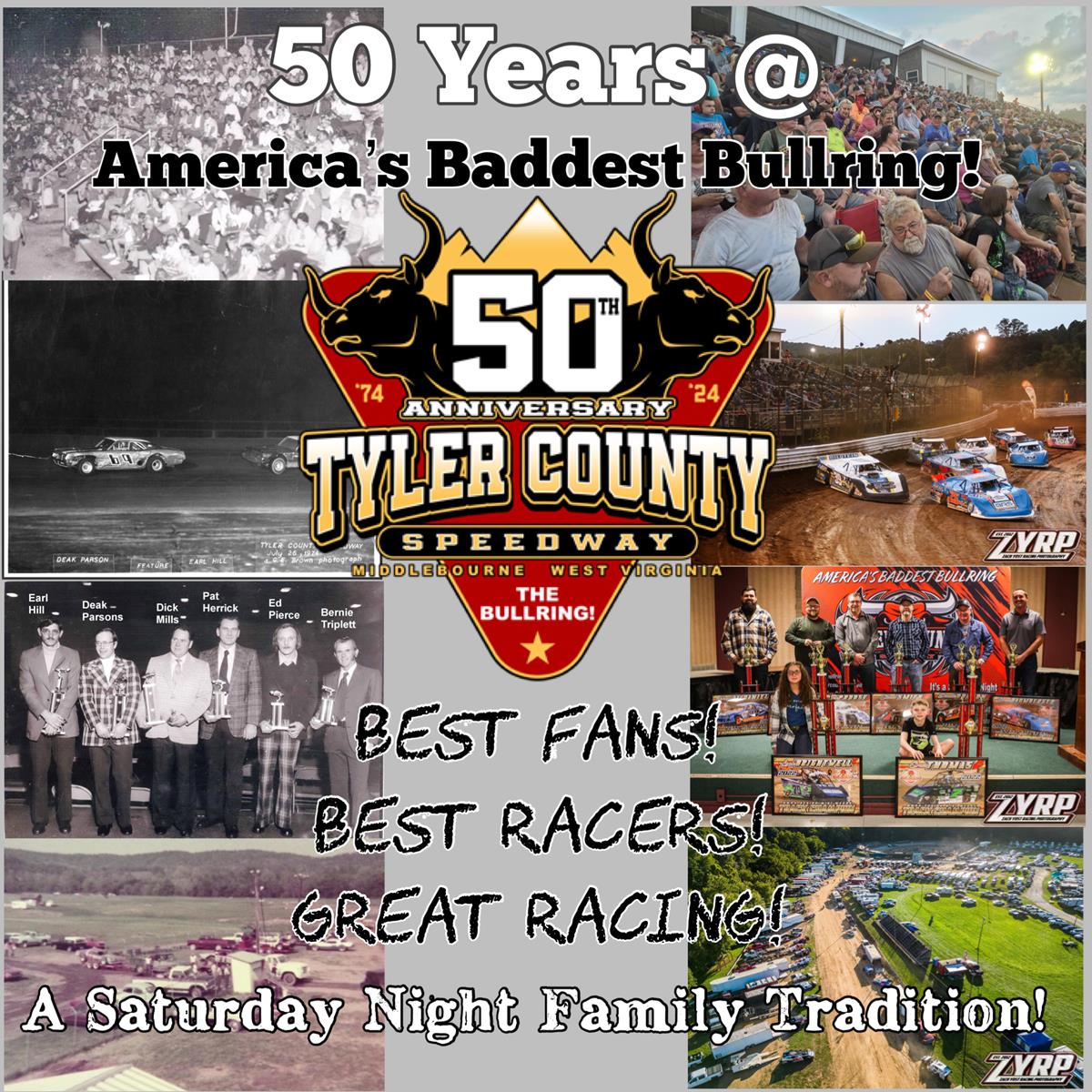The poster advertises the 50th Anniversary of the Tyler County Speedway, labeled "The Bull Ring." The layout comprises two columns of four pictures each, with a vertical gray rectangle in the center. Superimposed on this gray rectangle is the event's brand design featuring the numeral '50' with two bulls' heads extending from either side, and the words "50th Anniversary Tyler County Speedway" and "The Bull Ring" underneath.

The left column contains a mix of old black-and-white photographs and a faded color picture depicting historic moments, while the right column features vibrant, modern color photos. The images collectively showcase race cars in action, a full racetrack, enthusiastic crowds, and winners holding their trophies. Text on the poster celebrates "50 years at America's baddest bull ring" and highlights the event as "a Saturday night family tradition." Additional slogans emphasize the venue's reputation: "best fans, best racers, great racing." Sponsorship is noted with the mention of ZYRP, and the location is specified as Middleborn, West Virginia.